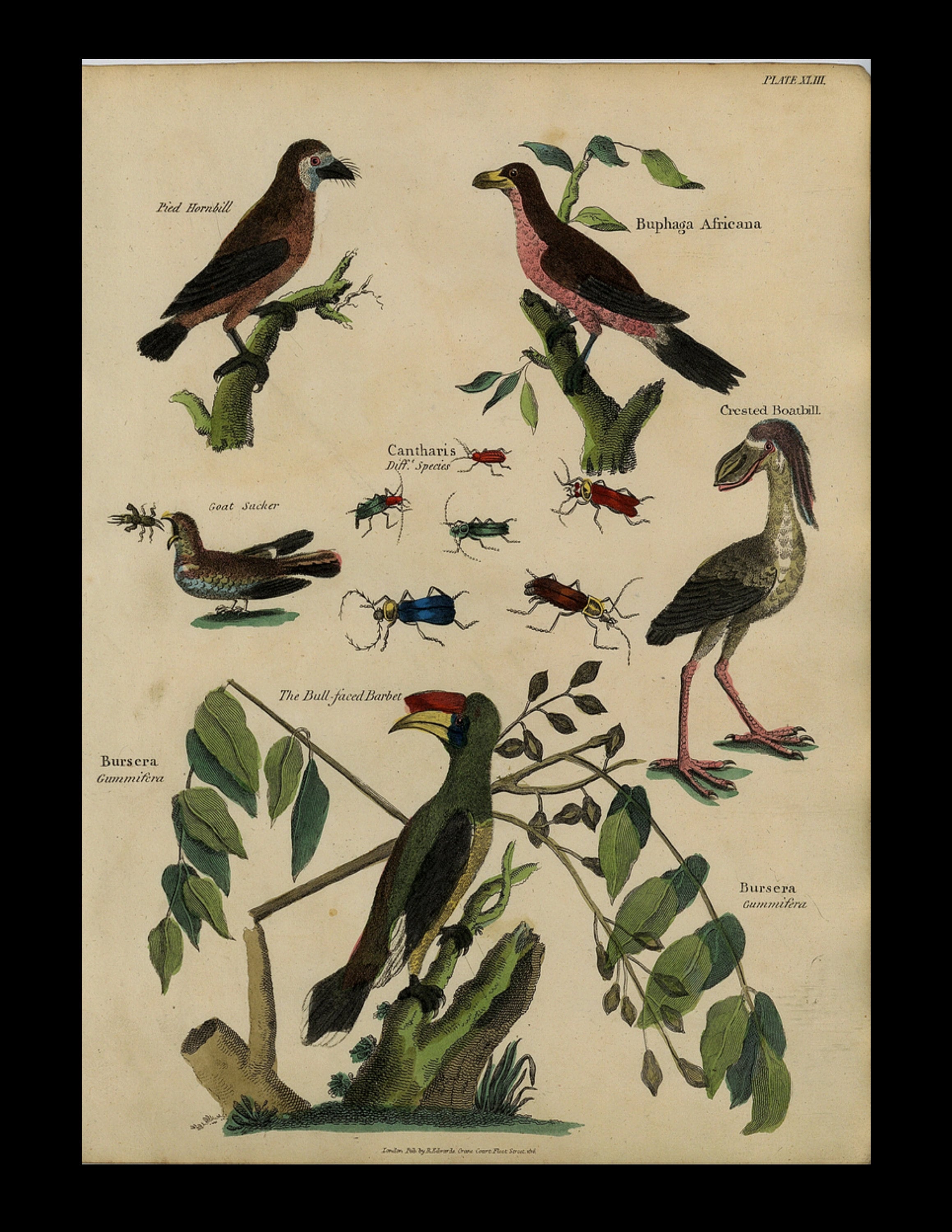This detailed and colorful scientific illustration showcases a variety of birds and insects meticulously arranged. The artwork features five distinct birds predominantly situated around the edges of the frame, which is black with beige matting. The bottom edge is graced by an illustrious parrot standing on a verdant plant. The parrot, dark gray to black with a yellow beak and red markings above, stands out against the foliage. 

Among the avian species are also a Pied Hornbill perched on a green stem to the right, identifiable by its brown and black plumage, and the Boufaga africana, a bird with a pink breast and brown feathers on another stem. There's a hornbill labeled 'crested boatbill' to the far right, resembling an egret with long, webbed, pink feet. Additionally, a duck-like bird labeled 'Great Sacker' appears, although details are slightly obscured.

In the center of the illustration, a diverse collection of six insects is vividly displayed. Among these are colorful specimens including blue, green, and burgundy bugs, named Catharis (C-A-N-T-H-A-R-I-S). The insects, characterized by long antennas, encircle the central bird arrangements.

Accompanied by Latin names, the illustration replicates the detailed style typical of scientific studies, with some textual elements and annotations at the bottom partially illegible, adding to the document's authenticity and charm. The birds, bugs, and scattered foliage, named Bursura, collectively create a rich tapestry of natural diversity.